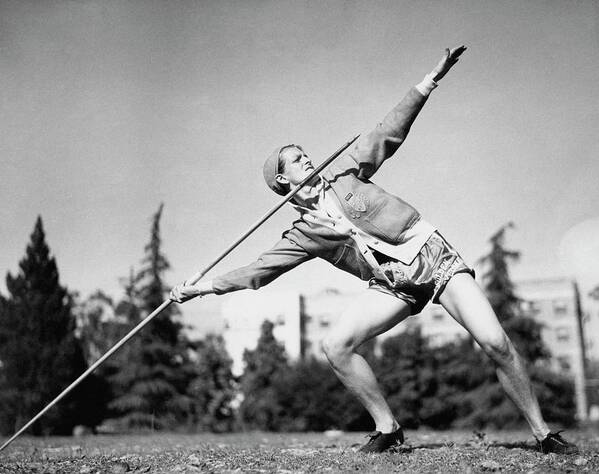In this black and white photograph, a javelin thrower—possibly a woman, dressed in what appears to be clothing from the 1920s or 1930s—strikes a dramatic pose. She is positioned on the right side of the image, leaning back with most of her weight on her right foot, her left foot barely touching the ground. Her right arm, taut and muscular, grips a javelin aimed at a 45-degree angle towards the upper right of the photo. Her left arm is raised, guiding the javelin’s trajectory. She is clad in very short athletic shorts, a cardigan, a cap, and possibly a leather jacket. The background reveals a cluster of tall, blurred pine trees and a distant, indistinct building under a very gray sky, enhancing the vintage feel of the scene.